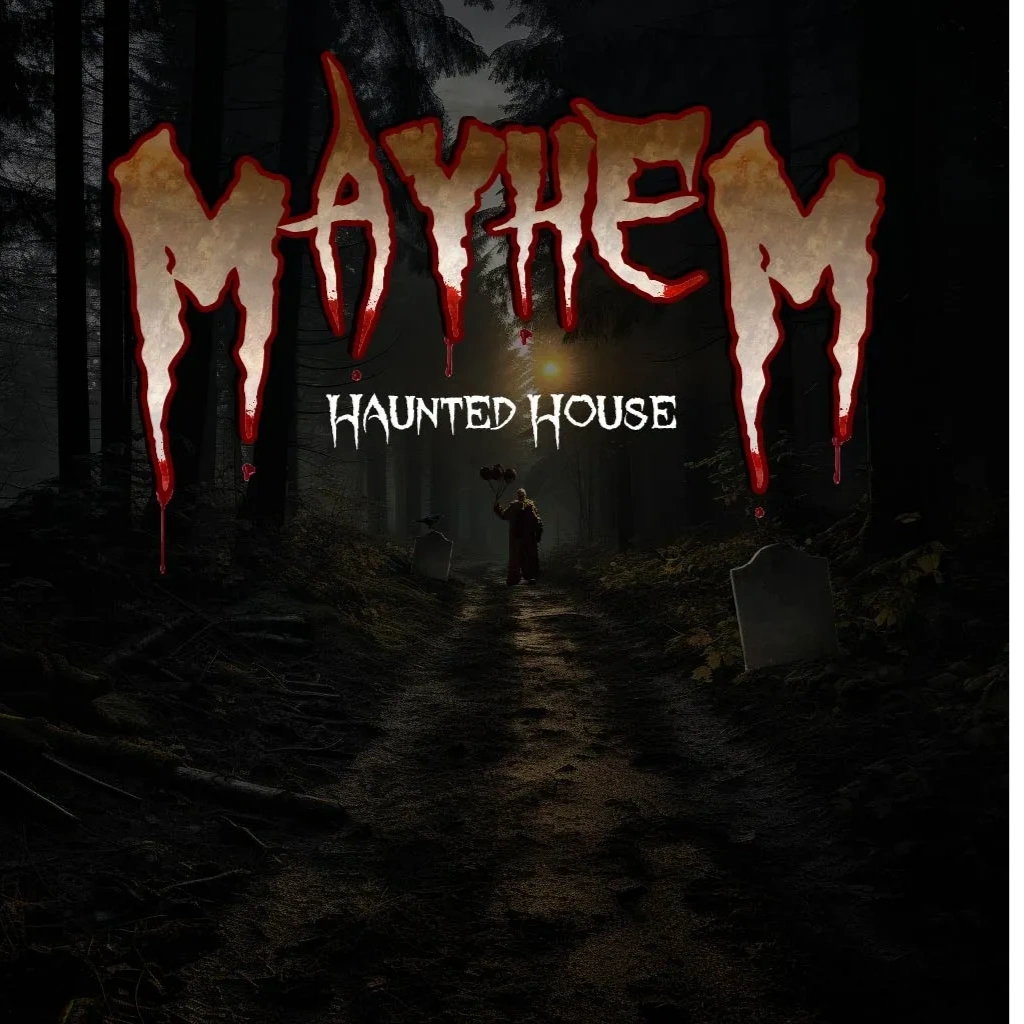The image appears to be an eerie poster or book cover, predominantly dark and foreboding in tone. Centrally, in stylized, torn-like capital letters, the word "MAYHEM" is prominently displayed at the top, with the off-white letters bordered in red, dripping blood from the edges. Below it, in a similarly unsettling font, is the subtitle "HAUNTED HOUSE." The scene unfolds along a muddy, debris-strewn path winding through a creepy, dense forest with grave markers flanking either side. The path is dimly lit by a setting sun or possibly a full moon, casting an ominous glow. At the end of the path stands a sinister clown, backlit to emphasize its menacing silhouette, which holds three balloons and appears to stare directly at the viewer, adding to the unnerving atmosphere.